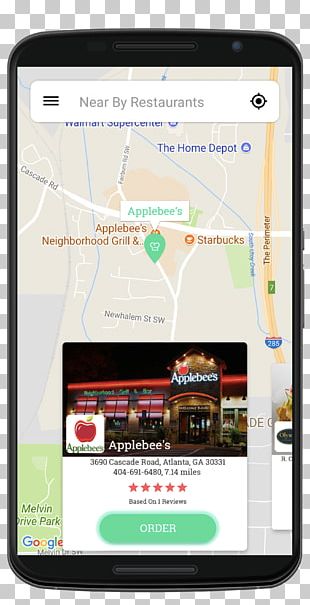This image features a cell phone displayed on a grey and white checkered background, suggesting it has been cut out from its original photo and placed on a transparent backdrop. The cell phone has a black border and is displaying the Google Maps application. Central on the screen, a pin marks the location of Applebee's on the map. Beneath the map, there is a detailed information box showing a picture of an Applebee's restaurant at the top. The bottom portion of this box contains the Applebee's logo on the left, the restaurant's name prominently displayed, followed by its address, star ratings, and a green "Order" button.

The map itself has a grey background, adding contrast to the screen's elements. At the top of the Google Maps interface, there's a search bar. On the left side of the search bar is a three horizontal line menu icon, and in the center, the text "nearby restaurants" is typed out. To the right, a location icon is visible, completing the typical layout of the Google Maps application interface.